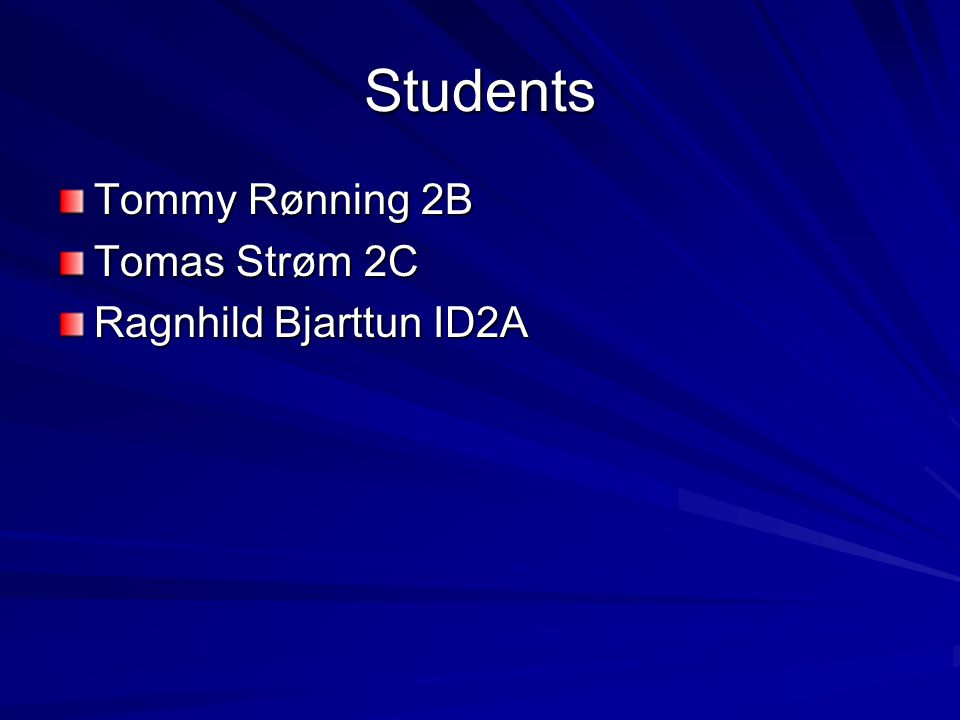An image resembling a PowerPoint slide features a blue background with various shades creating a light-ray effect, radiating horizontally from the right side. The background transitions from darker blue at the top left to a brighter blue at the bottom right. Positioned at the center top, the word "Students" is written in white text, predominately in lowercase except for the capitalized 'S'. Directly below, three bullet points list names: "Tommy Roening, 2B," "Thomas Strom, 2C," and "Ragnhild Jardin, ID 2A." Each bullet point is marked by a square that transitions from red on the left to white on the right. The text is in white font, and the lower half of the slide remains largely empty, showcasing the background design.